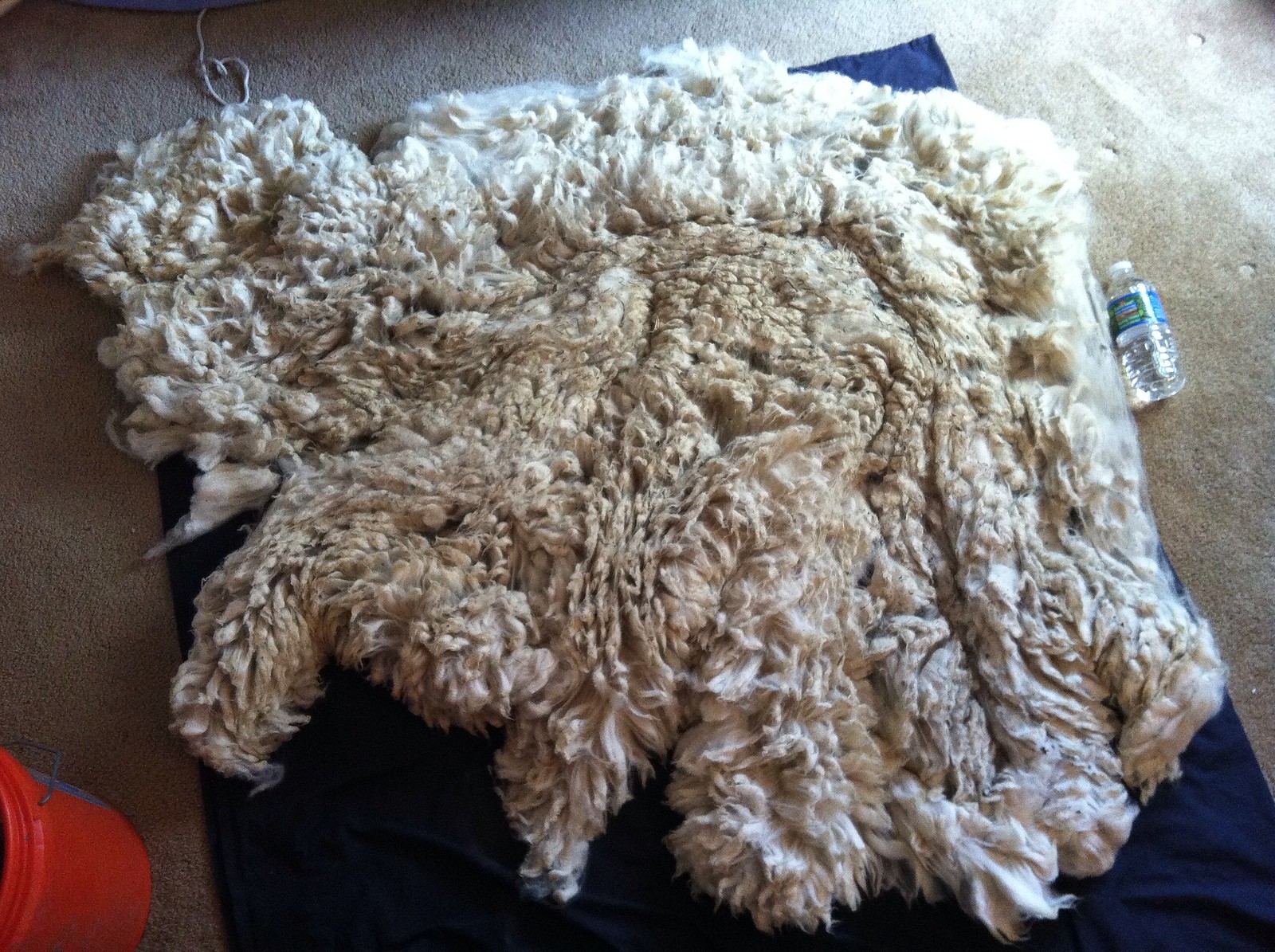The color photograph captures a large, irregularly-shaped mass of fleece or wool, reminiscent of a sheepskin rug, spread out on a wide blue towel. The fleece, slightly dirty and soiled, appears to have been freshly sheared, likely from a sheep that had some dirt or mud on its coat. Positioned on a concrete floor, the scene includes several objects to indicate the fleece's substantial size. To the right of the fleece lies a small 10-ounce plastic water bottle, while at the bottom left corner of the frame, a red five-gallon bucket is partially visible. The towel and fleece are laid out atop what seems to be a light grey or white carpet. The light source comes from the top left, making that area of the photograph the brightest, whereas the bottom left corner is noticeably darker. There are no people, animals, or vegetation present in the image.